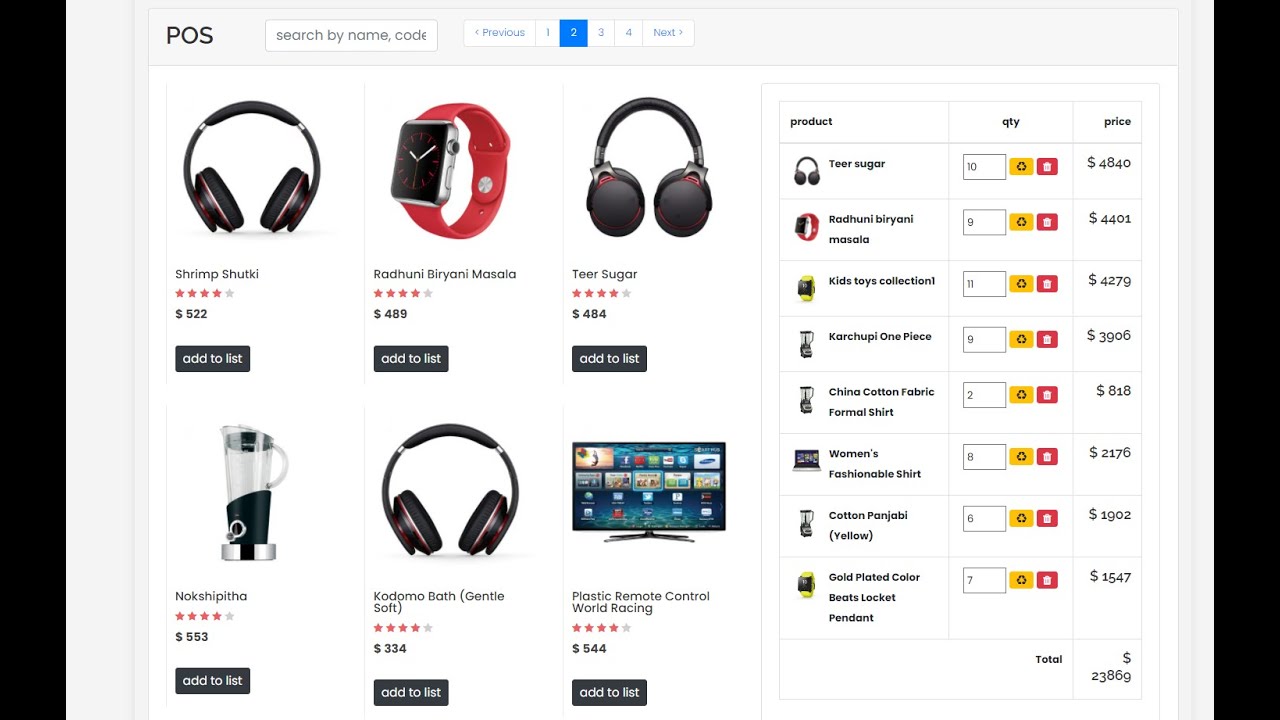The screenshot showcases a page from a website likely dedicated to selling various electronics and appliances. The website header features "POS" in the top left corner, with a search bar to the right prompting users to "search by name, comment code," although the full prompt is obscured. The screenshot reveals the user is browsing page 2, indicated by the highlighted "2" in blue among navigation buttons displaying page numbers 1, 2, 3, and 4, along with "previous" and "next" options.

Featured prominently at the top left of the page are black headphones named "Shrimp Shootkey," priced at $522, and rated four out of five stars. Positioned alongside, the "Red Honey Biryani Masala" smartwatch is listed at $489, also with a four-star rating. Further right, "Teen Sugar" headphones are priced at $484, sharing the same four-star rating.

In the bottom left, an item labeled "Nakshipita" appears as a blender or pitcher, costing $553. Adjacent to it, more headphones titled "Condomo Bath (Gentle Soft)" are priced at $334 and also rated four out of five stars. The bottom right features a "Plastic Remote Control World Racing" television, with a price tag of $544 and a matching four-star rating.

Beneath each product, there's an option to "add to list." The customer's cart displays a substantial quantity of items, including 10 Teen Sugar headphones, 8 Red Honey Biryani Masala smartwatches, 11 unspecified kids toy collection smartwatches, 9 Karchupi One Pieces, 2 China Cotton Fabric Formal Shirts, 8 Women's Fashionable Shirts laptops, 6 Cotton Punjabi Yellows, and 7 Gold Plated Color Beats Locket Pendants. The total cart value amounts to $23,869.